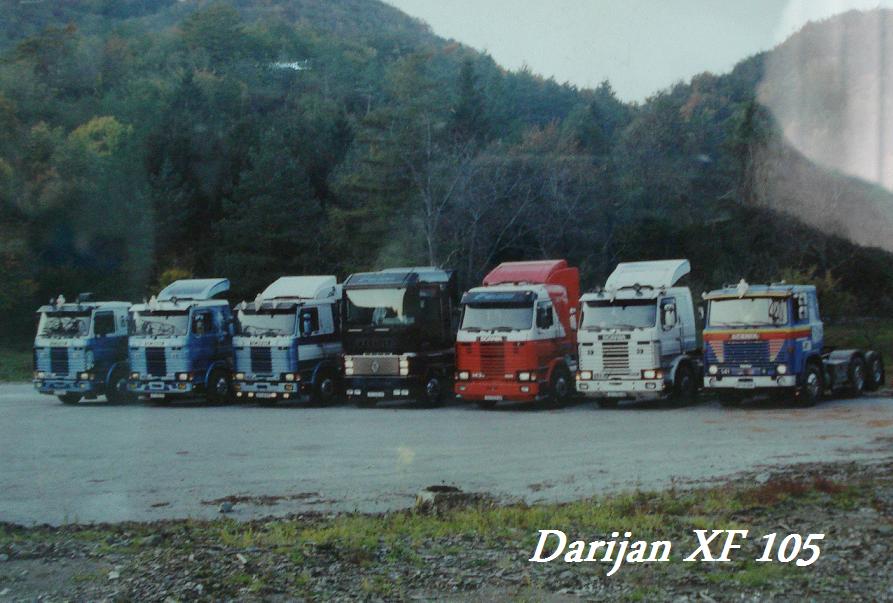The photograph showcases a lineup of seven old cab-over semi-trucks parked on an outdoor concrete parking lot. The trucks are positioned side by side, facing slightly to the left. Behind the trucks, there's a dense wooded area comprising both evergreen and deciduous trees, while the foreground features a rocky, scrubby grass area with sparse vegetation. The semi-trucks come in various colors: from left to right, there is a solid blue cab, a light blue cab, a blue cab with white accents, a black cab, a red cab with white outlining, a white cab, and a blue cab with orange and yellow stripes. The asphalt parking lot appears slightly wet, suggesting it might have recently rained. In the lower right-hand corner of the image, the text "Darajan XF-105" is visible, indicating the model or series of the trucks.